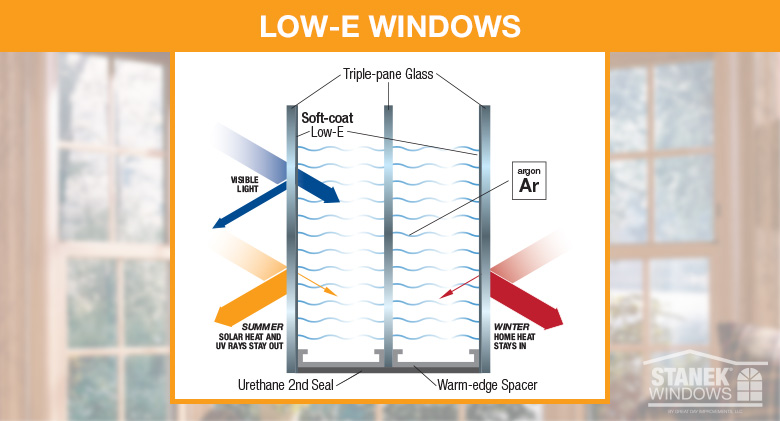This image is a detailed schematic for Low-E Windows, depicted on a horizontally oriented photograph with a whitewashed background of house windows. At the top is a bold orange strip with "LOW-E WINDOWS" written in white uppercase letters. Below this strip is a white section illustrating the technical aspects of the window. The central schematic features a vertical, silver-framed window drawing with the top frame open. 

The window's design elements are meticulously labeled: 
- "TRIPLE PANE GLASS" is indicated with arrows pointing to the outer frames.
- "SOFT-COAT" followed by "LOW-E" is noted in the top left section of the window.
- "AG" or "Ar" (possibly indicating argon gas) is featured nearby.

Arrows around the silver frame suggest the movement of different types of air: 
- A gradient blue arrow for cool air in the upper left,
- A gradient yellow arrow for warm air in the lower left,
- A gradient red arrow likely showing heat flow on the right.

Additional features are highlighted with labels and arrows pointing to parts of the frame:
- "URETHANE SECOND SEAL" on the left,
- "WARM-EDGE SPACER" on the bottom right.

In the lower right corner, the logo for STANEC Windows is displayed, with "STANEC" in bold white letters and "WINDOWS" in a smaller, narrower font, accompanied by an atrium window symbol above the text. The illustrative and descriptive elements communicate how the window effectively blocks UV rays, solar heat in summer, and retains home heat in winter, enhancing energy efficiency.